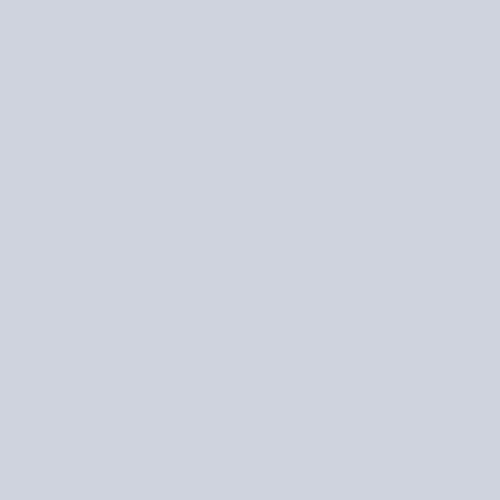A square, battleship-gray box is depicted in the image, offering a versatile canvas for a myriad of purposes. Its simple, monochromatic design can effortlessly accommodate a photograph, a poem, or any form of written content. Imagine transforming this space into the introductory page of a pamphlet, perhaps showcasing popular restaurants with visually appealing images of their signature dishes taken by food enthusiasts. Alternatively, it could serve as a detailed, pictorial guide on car maintenance and repairs—a practical resource for DIY aficionados. For the academically inclined, the box could feature educational snippets, such as the mechanics of earthquakes, offering a concise, informative overview of seismic activity and its causes. This understated gray box holds endless potential for creativity and information-sharing.